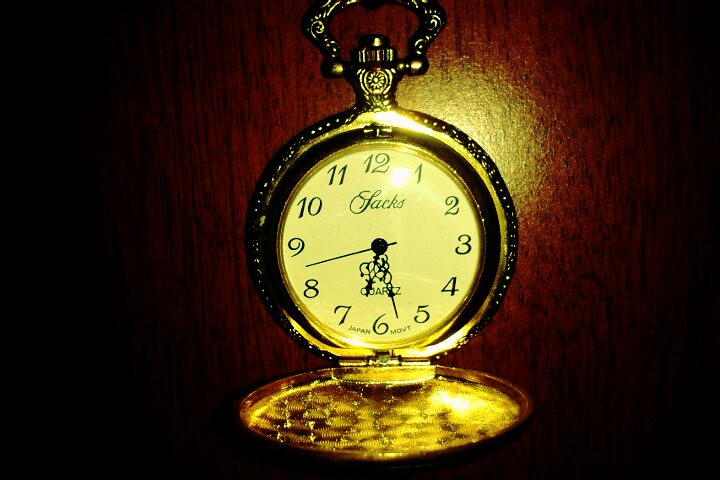This detailed photograph features a vintage gold pocket watch resting on a richly varnished wooden surface. The watch is captured in a close-up shot using flash photography, highlighting its intricate details. The circular gold cover, or hatch, is open and pointed outwards, revealing the white analog clock face. At the top center of the dial, the word "SACS" or "JAX" is inscribed in an elegant script font. The watch face includes ornate hour and minute hands as well as a second hand. Near the bottom, small text reads "Japan MOVT" and indicates that it is a quartz watch. The pocket watch has a finely designed gold border around its housing and features a winder button and a small piece at the top for attaching a chain. The time displayed on the watch is approximately 6:27 and 43 seconds.